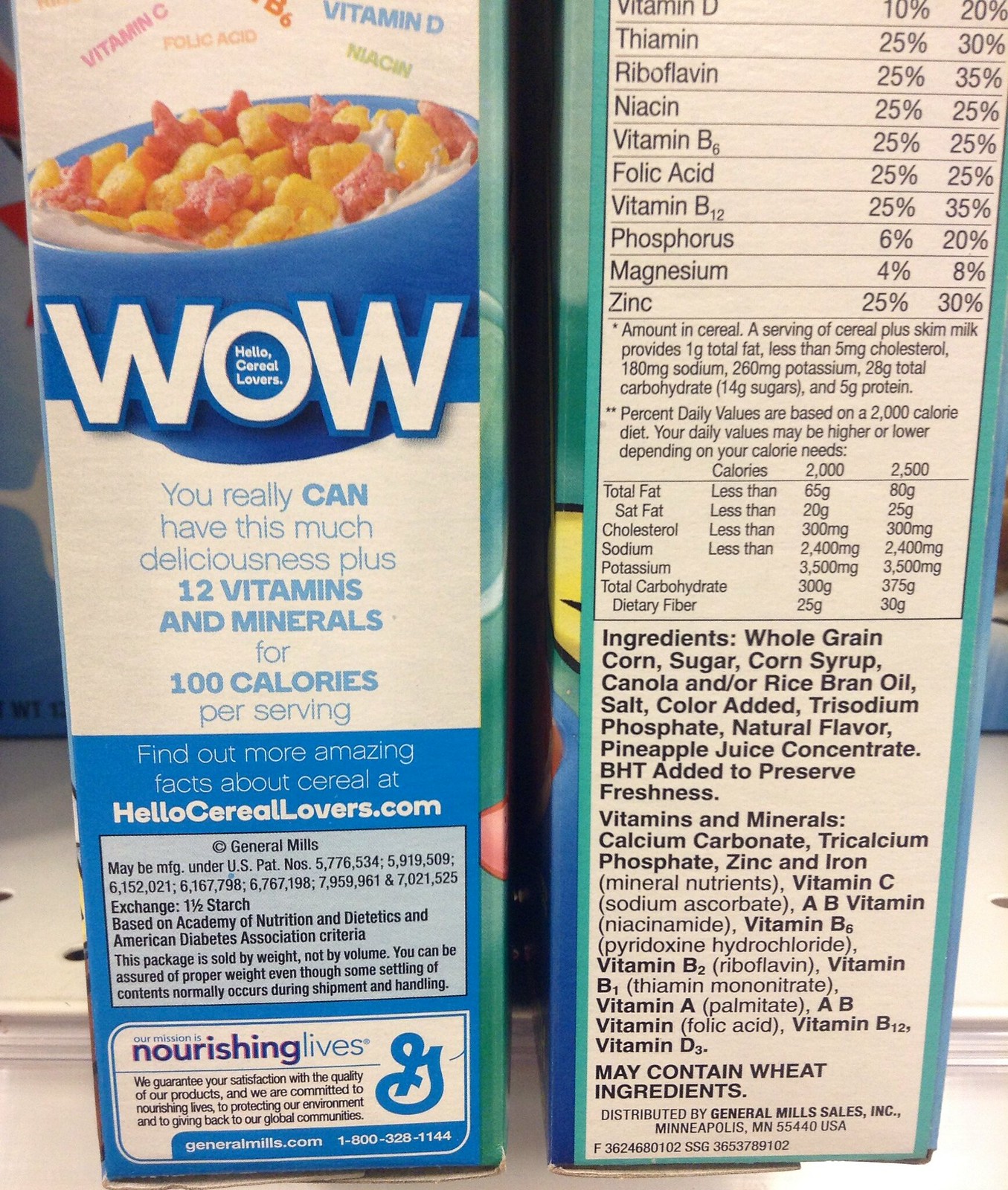This image depicts two cereal boxes positioned on a white shelf in a retail store, with other similar boxes faintly visible in the background. Both boxes are of the same cereal, shown from different sides. The box on the left prominently displays a photograph of a blue bowl filled with golden square pillow-shaped cereal pieces and red star-shaped pieces, reminiscent of Captain Crunch. Across the bowl in bold white letters, it says "WOW," with the words "Hello Cereal Lovers" inside the 'O'. Below this, the text details that you can enjoy this delicious cereal with 12 vitamins and minerals for just 100 calories per serving. Further down, in white letters on a blue background, it invites consumers to "Find out about amazing facts about cereal at HelloCerealLovers.com." At the bottom, it includes a statement and information from General Mills, ending with the phrase "nourishing lives." The box on the right focuses on nutritional information, listing the various vitamins, minerals, and ingredients included, along with detail on potential allergens. Both boxes extend from the top to the bottom edges of the photograph, emphasizing their prominent shelf presence.